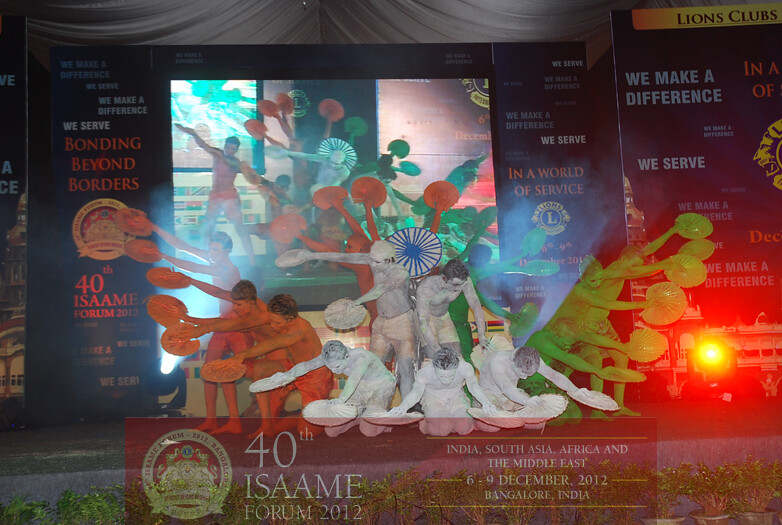The image showcases a vibrant and colorful stage performance at the 40th ISAME Forum 2012, held from December 6th to 9th in Bangalore, India. The dancers, painted in solid colors—white in the center, green on the right, and orange on the left—are dramatically arranged to resemble the spread wings of a bird. They each hold round, Asian-style fans, and some have fans raised above their heads. The stage is backed by a large billboard displaying a live screen of the performance, enhancing the visual spectacle. The backdrop and signage emphasize themes such as "Bonding Beyond Borders in a Service World" and "We Serve," highlighting the event organized by the Lions Club for regions including India, South Asia, Africa, and the Middle East.